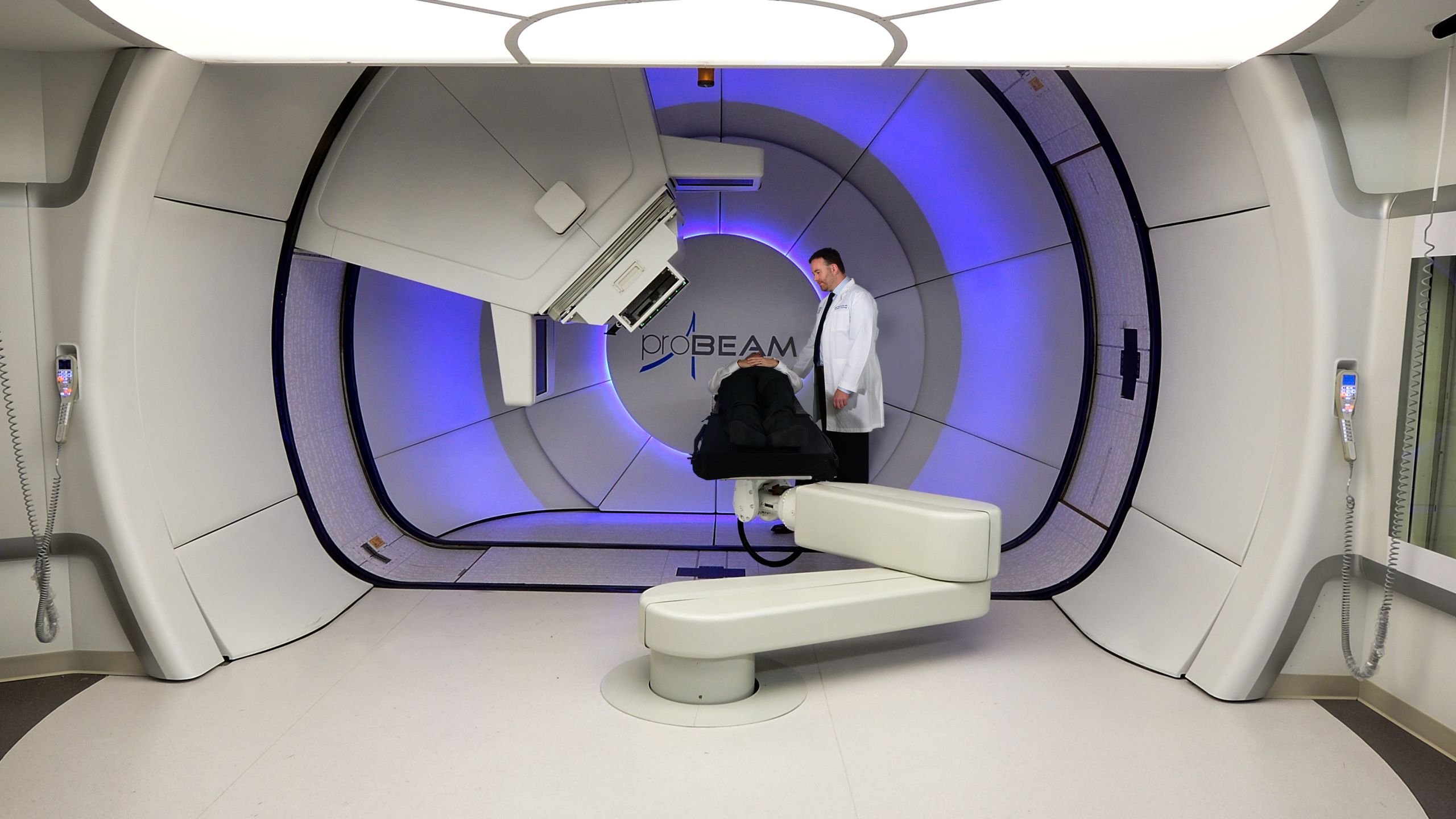The photograph captures a futuristic medical imaging center illuminated by artificial light. Dominating the scene is a large, high-tech diagnostic scanner identified by the word "PROBEAM" glowing in blue neon atop a circular chamber built into the back wall. At the center of the image is a patient reclining on a bed outfitted with a robotic arm capable of swiveling and maneuvering to various positions, suggesting advanced imaging capabilities. The patient is dressed in black pants and a white shirt, with hands folded on his belly, covered by a heavy-duty blanket. Positioned nearby is a doctor or scientist dressed in a long white lab coat, attentively standing over the patient. The intricate scanner, larger than a CT scanner and resembling a futuristic space chamber, features multiple arms and lenses extending and protruding from various angles, aiming at the patient and capturing detailed images. The room is brightly lit, enhancing the clean, sterile, and technologically advanced atmosphere.